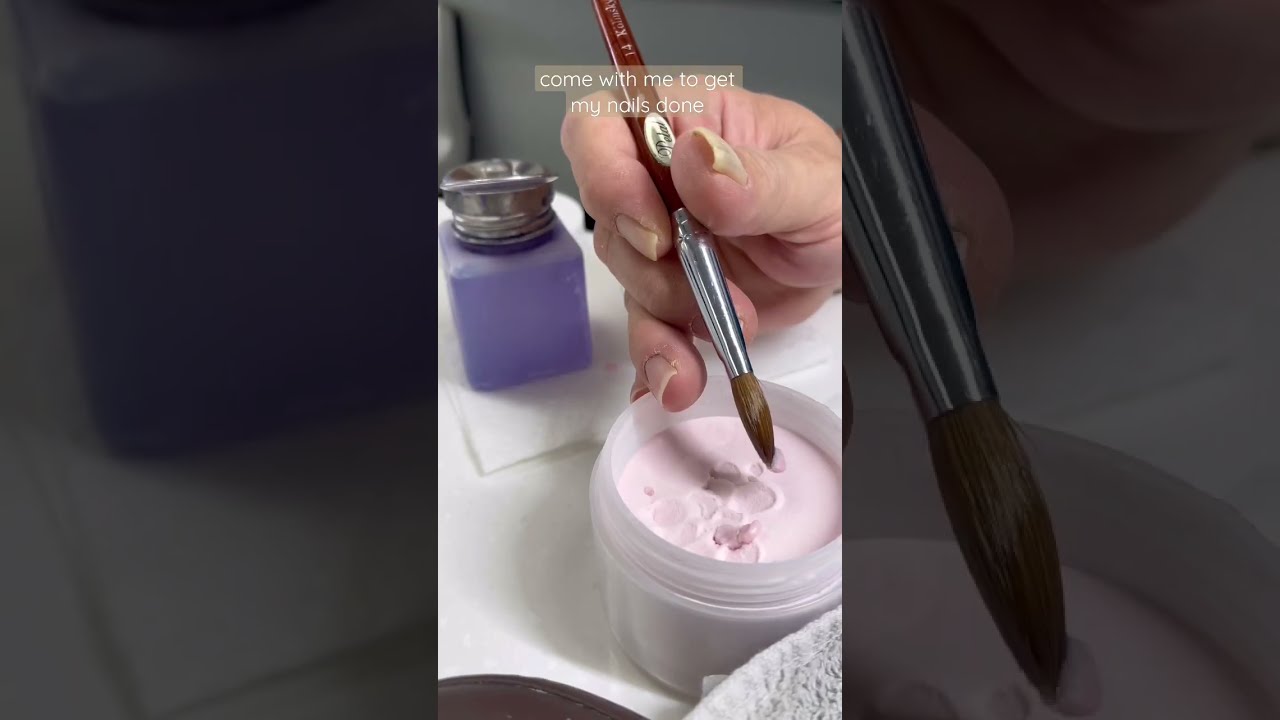The image is a horizontal triptych composed of three equal-sized panels from left to right. In the left panel, there is a dimly lit view featuring the upper portion of a purple jar with a silver top, partially cut off on the right side. Beneath the jar, the rest of the panel is darkened. Moving to the middle panel, it's brighter and showcases a woman's hand of light skin complexion, holding a brush and dipping it into a white jar filled with a substance that might be nail-related or a thick cream. The brush has brown bristles with a silver ferrule, and the scene is set against a lightly colored surface that resembles a white vanity table. The woman's slightly long nails are noticeable, and behind her hand, you can see the aforementioned purple jar with white writing across the top that reads, "Come with me to get my nails done." In the background, below this layer, there's a darker image adding depth to the scene. The right panel is a close-up of the same brush from the middle panel, showing the brown bristles and the person's hand holding it. This panel is also darkened, making it slightly harder to view details, but the round jar and the substance inside are still visible as the brush dips into it.